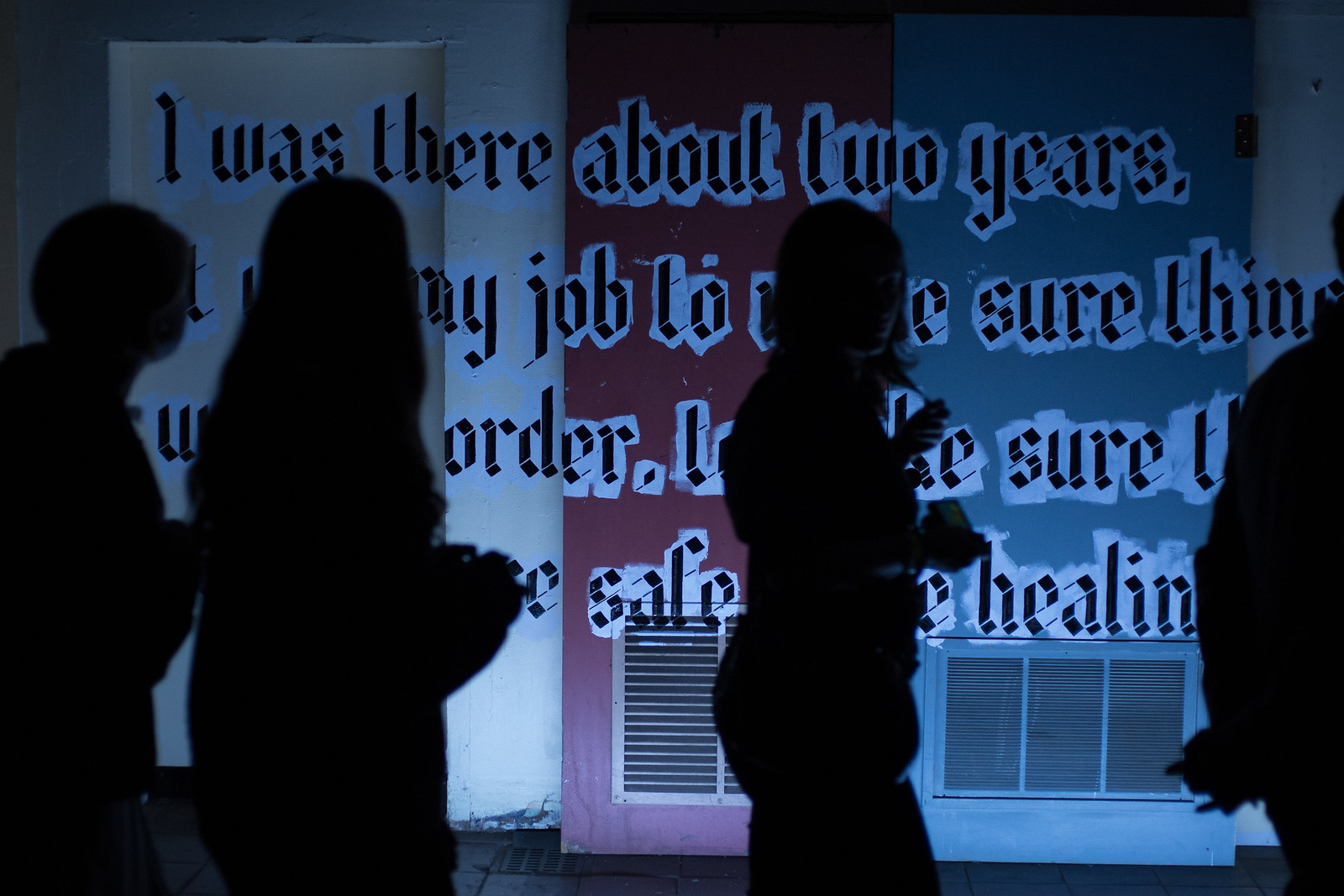In this rectangular indoor photograph, we see the shadowy silhouettes of four individuals walking from left to right in a single file line. The figures are predominantly black, with a faint blue light outlining their forms, and the details about them are largely obscured. However, the two central figures appear to be female, discernible by their body shapes and long hair, while the gender of the person on the far left is tentative as male. The person on the far right is partially cropped and indeterminable.

The backdrop is an old, cracked, plastered wall painted in vertical stripes of yellow, red, and blue hues. A doorway is also visible within the image, integrated into the painted and graffiti-covered wall. The graffiti consists of black lettering with a white outline, sprawled across the different colored sections and a vent below. Though the text is partially obscured by the walking figures, some legible phrases include: "I was there about two years," "Job 2 Sure," "Order Sure," and "Safe Healing."